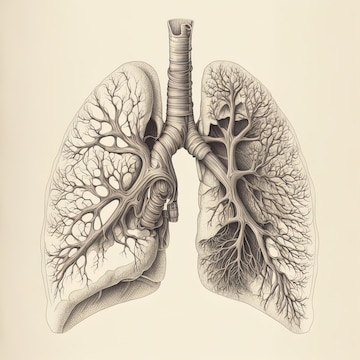This detailed vintage-style illustration, likely from an old medical textbook, depicts a pair of human lungs meticulously drawn in pencil or charcoal on beige-tinted paper. The diagram showcases the stark contrast between the left and right lungs. The left lung is clearer, free of congestion, and demonstrates fewer veins, making it appear less obstructed. In contrast, the right lung is heavily congested, with veins and capillaries densely branching out, almost resembling intricate tree branches, inhibiting its expansion. The rendering is three-dimensional, with shading that enhances its depth. The lungs are connected centrally by a trachea that extends upward but cuts off before the edge of the image. The detailed depiction aims to highlight the structural and functional differences between a healthy and a congested lung.